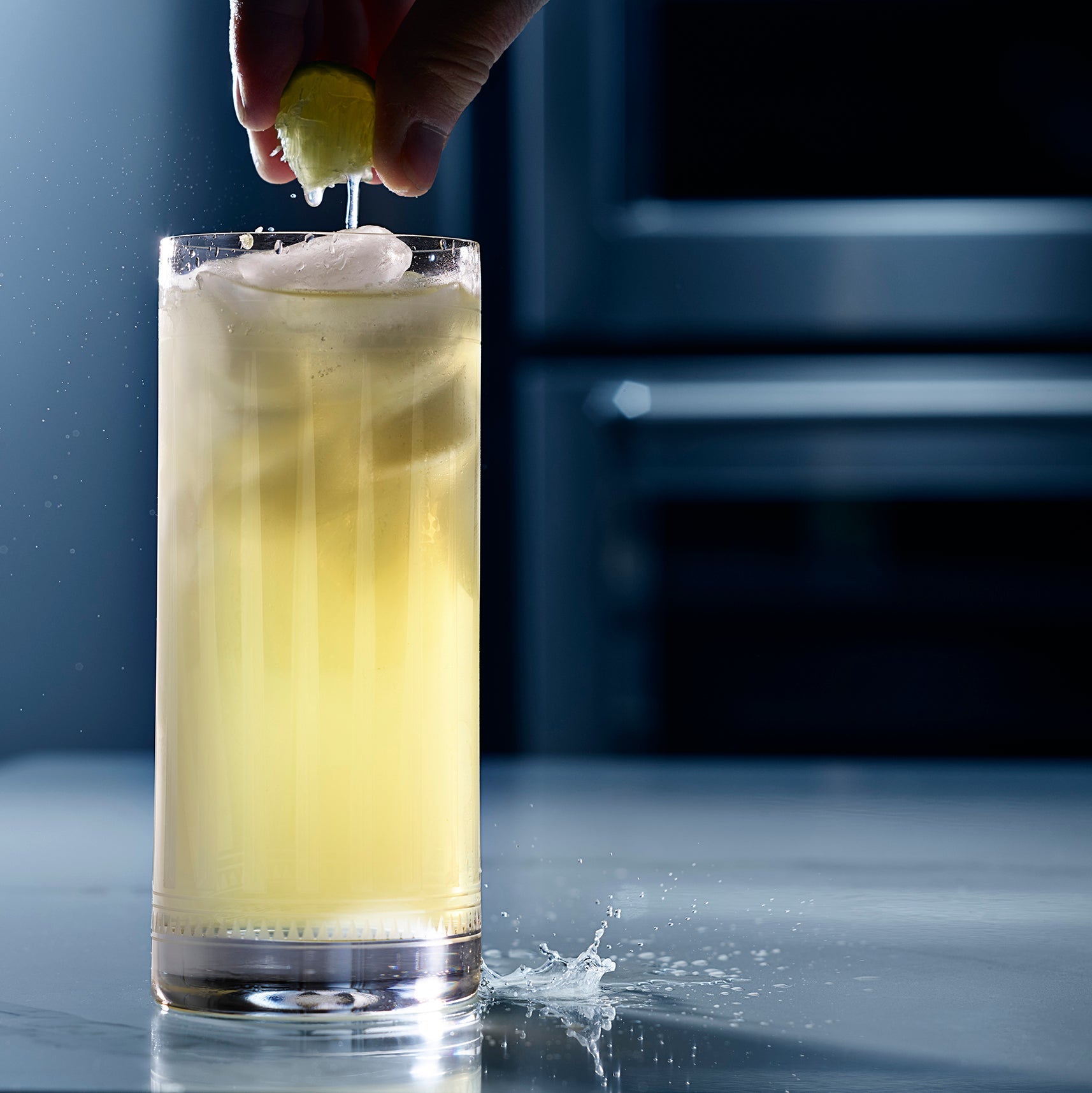In a dimly lit kitchen, a close-up photograph captures a hand squeezing a lime into a tall, clear highball glass brimming with pale yellow lemonade. Ice cubes float at the top of the drink, and a few droplets of juice can be seen splashing onto the glossy, white surface below. The background features blurred, stainless steel appliances and a dark blue wall, which contrasts with the light yellow of the lemonade. The scene is centered around the glass, positioned slightly left of center, emphasizing the freshness and vibrant colors of the drink amidst the subdued, shadowy kitchen setting.